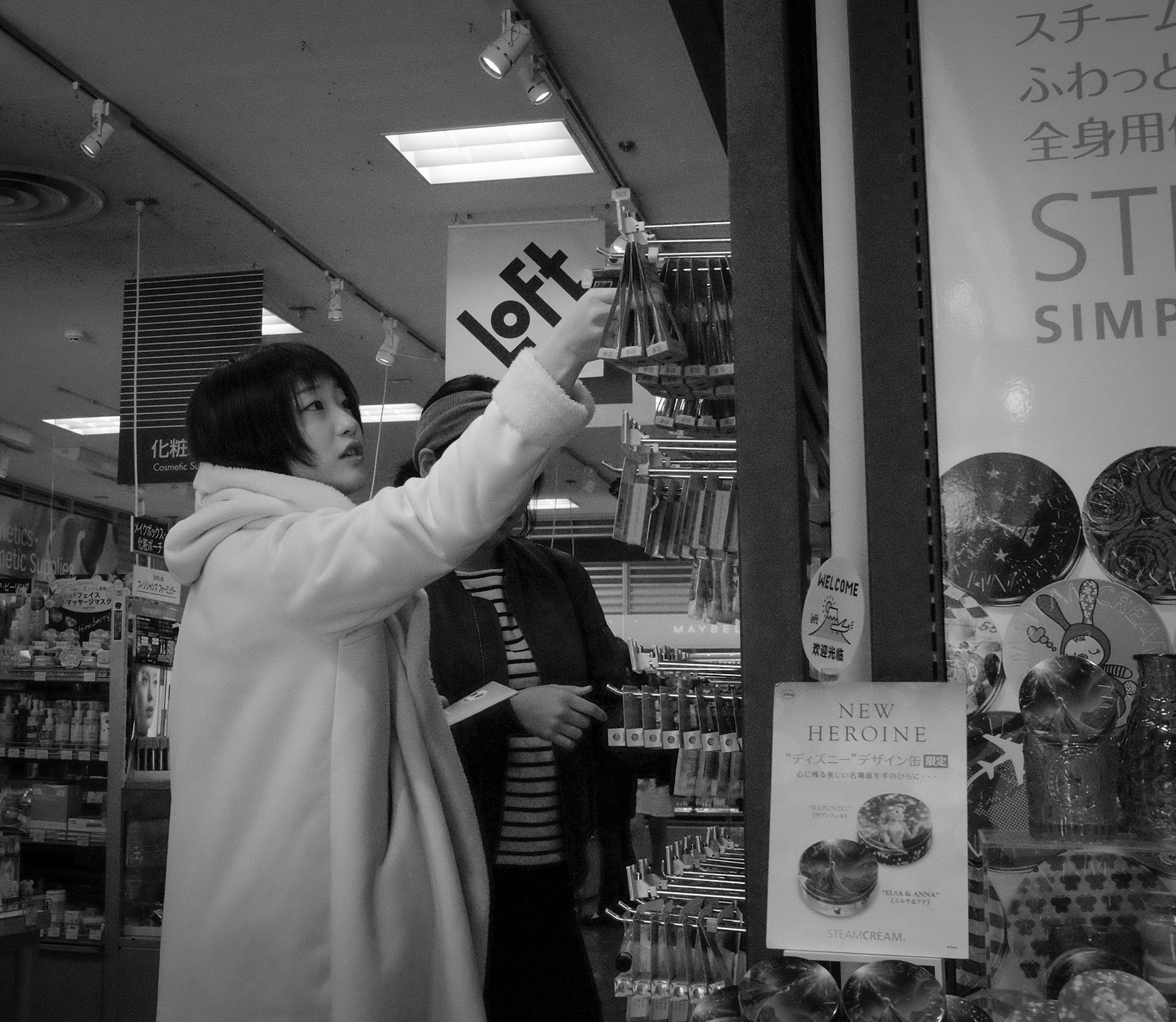In this square-shaped black and white photograph, we see an indoor shop featuring a couple of women standing centrally in front of a wall laden with racks of small products, likely cosmetics in small boxes, hanging from metal pegs on perforated boards. One woman is prominently reaching up to take a product off the top shelf. She is wearing a distinct long white hooded coat, obscuring the face of another woman standing slightly behind her. This second woman is dressed in a black jacket over a black and white striped shirt. The store's interior includes several banners hanging from the ceiling; one notably has the word "loft" written diagonally in English, while another exhibits a pattern of black and white lines with Asian script underneath. The shop appears cluttered with various items and utensils displayed on shelves, creating a busy atmosphere accentuated by mirrors and lights at the top of the frame. Signage throughout the store is predominantly in an unidentifiable Asian language, adding an international essence to this detailed depiction of a retail environment.